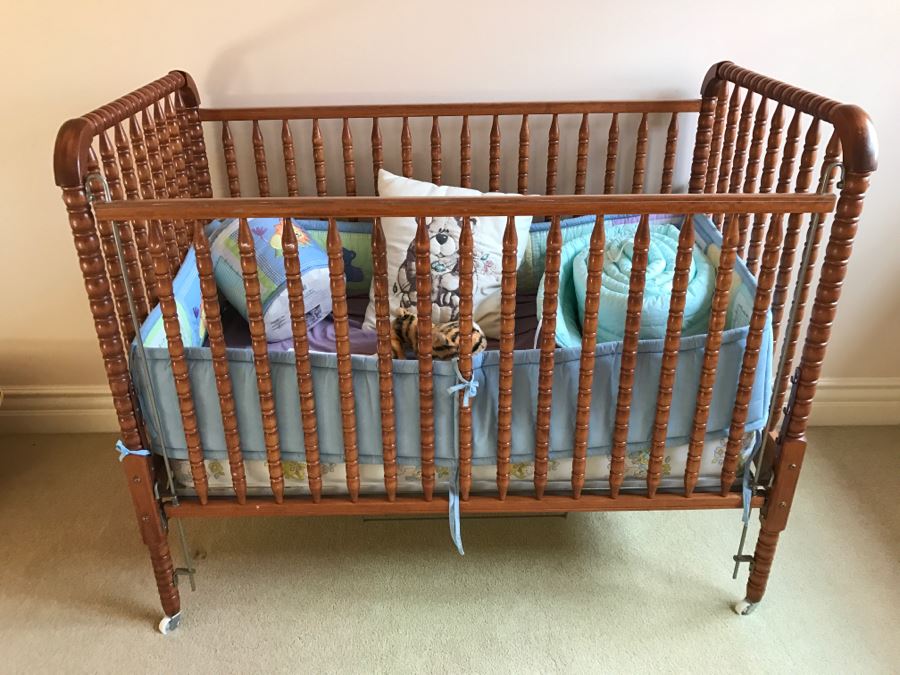The photograph captures a detailed scene of a vintage-styled, rosewood crib positioned inside a warmly decorated room. The room features a light greenish-gray carpet and beige cream-colored walls, creating a soothing atmosphere. The crib's ornate carved pattern adds an element of sophistication and charm. Inside the crib, a blue lining provides a soft and comforting base, complemented by various cushions and pillows, including a central white pillow adorned with a bear design. A couple of blankets are neatly rolled, enhancing the made-up look of the crib. Adding a touch of whimsy, a plush tiger toy sits prominently in the foreground. The crib, which is currently vacant, rests on small wheels, indicating its mobility. This well-arranged scene emphasizes the crib's readiness and inviting nature.